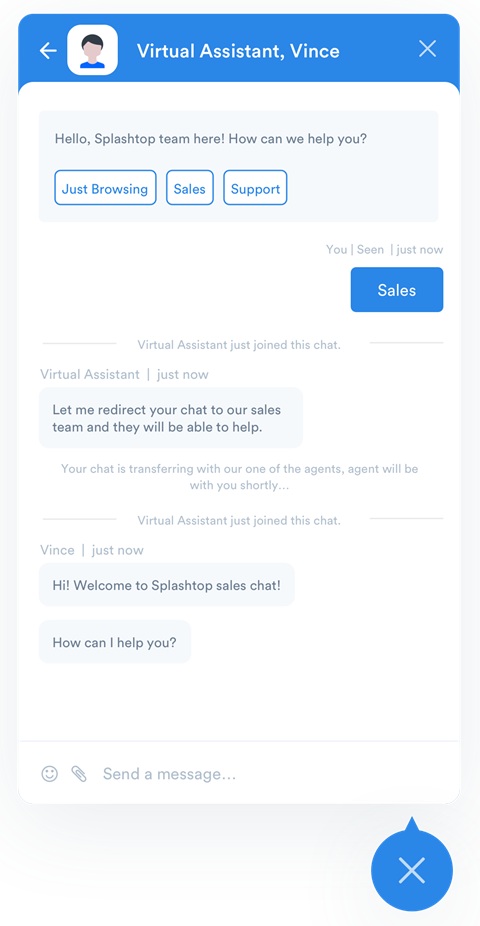This screenshot depicts the user interface of a mobile application, likely for customer support, identified as the Splashtop app. The top of the screen features a blue header with a generic male cartoon avatar without a facial representation, labeled as "Virtual Assistant Vince," flanked by an "X" symbol to close the session.

Beneath the header, a dialogue box from Vince states, "Hello, Splashtop team here, how can we help you?" Users are offered three response options: "Just browsing," "Sales," and "Support." The interface indicates the virtual assistant's last active time with phrases like "just now." The user selected "Sales," prompting Vince to respond, "Let me redirect your chat to our sales team, and they will be able to help." Subsequently, a smaller text informs the user, "Your chat is transferring with one of our agents, an agent will be with you shortly."

However, the interaction does not progress to a live agent. Instead, Vince reappears, stating, "Hi, welcome to Splashtop sales chat, how can I help you?" The bottom of the screen contains an input field with icons for inserting emojis, attaching files (represented by a paperclip), sending messages, and another option to exit the chat.

Overall, the screenshot captures the automated nature of Splashtop's AI-driven customer support, highlighting its initial engagement process and visual elements of the mobile app interface.